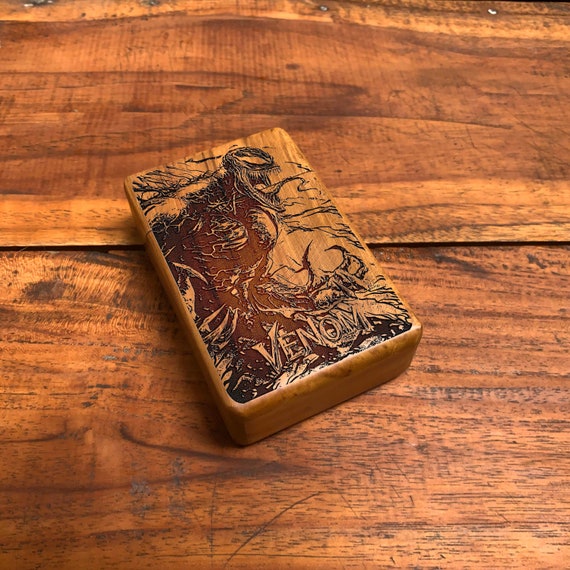Resting on a medium brown, scratched wooden table is a small, mahogany-colored rectangular wooden block, roughly 1 inch wide and 3 inches long. The block features a detailed carving and painting of Venom, the iconic character from the Spider-Man universe, with his menacing open mouth, sharp teeth, and large eyes. Venom's characteristic tendrils or strings are faintly depicted around him. At the bottom of the block, "Venom" is clearly etched. There is a thin black horizontal line visible along the wooden table's surface where two sections meet, marked with nails. The entire scene, including the block and the table, shares a cohesive brown hue with intricate textures, giving it a rustic appearance.